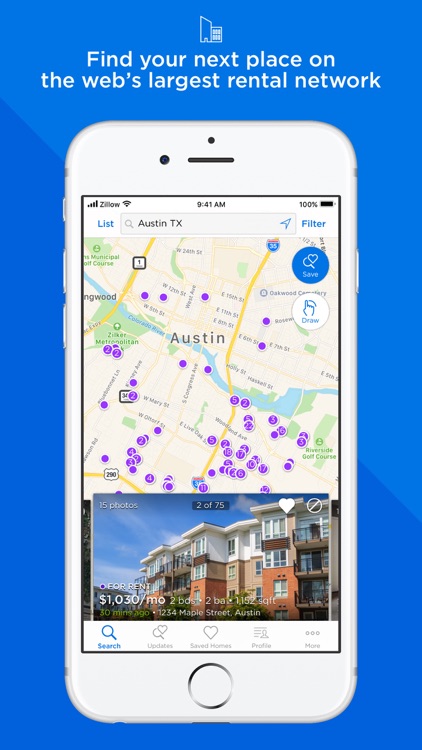The image features a blue screen with the text "Find your next place on the web's largest rental network" prominently displayed at the top. Below this text, a white smartphone is depicted. The phone has noticeable buttons along its side, including a circular button at the bottom center.

On the phone's screen, a map of Austin, Texas is displayed. At the very top of the screen, the name "Zillow" is visible in the white header area, along with reception, WiFi symbols, battery status showing 100%, and the time. Below the header, there is a search bar containing the text "Austin, Texas."

The map itself is dotted with numerous purple markers indicating various property locations. A river runs through the center of the map, and detailed road markings include yellow lines and a shield symbol indicating Interstate 35 (I-35). On the lower part of the screen, a listing stands out with an image of an apartment building. The listing states "For rent: $1,030/month, 2 bath, 2 bedroom, 1,152 sq ft," showcasing a multi-story building with white, brown, and orange façade.

At the very bottom of the phone's screen, five navigation icons are visible, labeled as "Search," "Updates," "Saved Homes," "Profile," and "More."